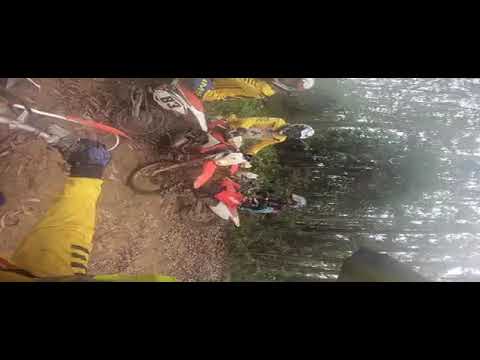The image depicts a sideways view of an outdoor scene in the mountains, featuring three motorcyclists on dirt bikes. The photo is slightly blurry, making some details unclear. All the riders are facing the camera, riding red and white motocross bikes. The first bike displays the number 83. Two of the riders are clad in bright yellow jackets with white helmets, while the third biker, positioned at the far end, is wearing black. In the foreground, an arm dressed in a yellow sleeve with a black glove is seen gripping a handlebar, likely belonging to the person taking the picture. The background reveals a densely wooded area with tall, skinny trees, suggestive of a mountain setting. Sunlight filters through the foliage, indicating it is daytime. The entire scene is set on a brown dirt path.